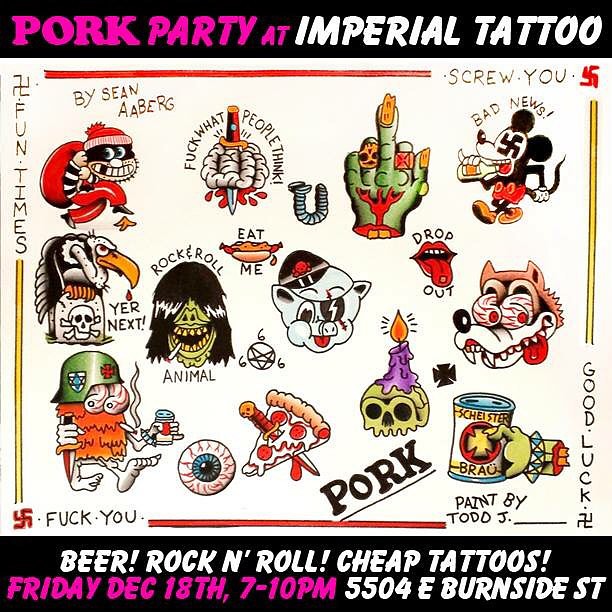This visually striking advertisement for a tattoo party features a collection of eclectic and colorful tattoo designs set against a cream-colored background. Topping the image, a black banner with vibrant pink and white text announces "Pork Party at Imperial Tattoo." Below, an array of unique tattoos is showcased in various vivid colors including reds, purples, greens, blues, yellows, and blacks. The designs range from playful to rebellious, with images such as a pizza with a knife, a skull with a candle, an eyeball, a robber carrying a sack, a zombie hand with the middle finger raised, Mickey Mouse, a wolf, and slogans like "Rock and Roll Animal" and "Drop Out." These tattoos are arranged in a grid-like pattern. At the bottom, another black banner proclaims the event details in white and pink text: "Beer, Rock and Roll, Cheap Tattoos, Friday, December 18th, 7-10 p.m., 5504 East Burnside Street." This bold and lively promotional image clearly advertises a dynamic and edgy tattoo party event.